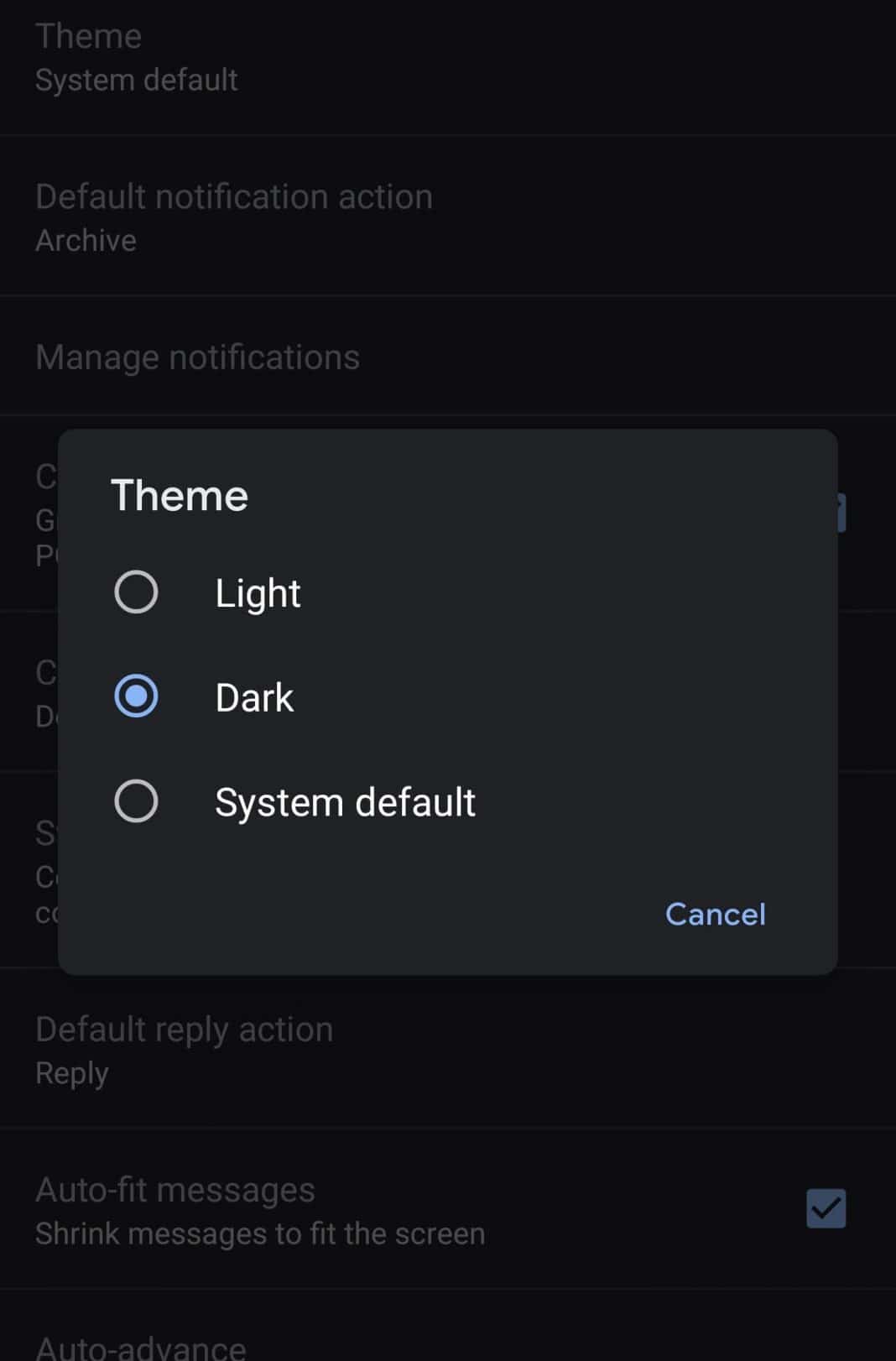The image is a screenshot, possibly from a larger smartphone, with a predominantly black background and a pop-up menu in the middle. The background text is in a darker shade of gray, adding to the dark theme aesthetic. At the top left corner of the screen, the text reads "Theme," followed by "System default" directly underneath, all left-justified. Below these, the options listed sequentially are "Default notification action," set to "Archive," and "Manage notifications."

The central feature of the screenshot is the pop-up menu, which partially obscures some text below it. However, beneath the pop-up, the visible text includes "Default reply action," set to "Reply," and, at the very bottom, "Auto-fit messages," with a description "Shrink messages to fit the screen," alongside a checked checkbox on its right.

The pop-up box itself is labeled "Theme" and offers three clickable bubble options labeled "Light," "Dark," and "System default." The "Dark" option is selected, indicating the user's current preference. Additionally, at the lower right-hand corner of the pop-up box are options for "Cancel" and "OK" in blue, affirming the choice for the dark theme.